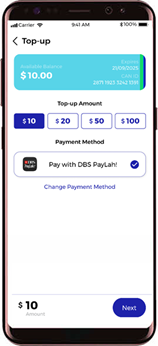This image features a close-up of an iPhone screen displaying a payment application interface. The application’s title, "Top Up," is prominently shown at the top of the screen. Directly beneath the title is a blurred blue box where the primary information, including a confirmed payment amount of $10, is visible. Below this section, users can select a top-up amount from four preset options: $10, $20, $50, and $100. Further down, in the payment method section, the only available option listed is "Pay with DBS PayLah." At the bottom of the screen, a prominent blue "Next" button is provided, enabling the user to proceed with the payment process.